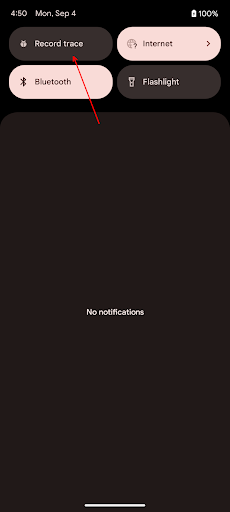The image depicts a smartphone screen displaying several key elements. At the top of the screen, the time is shown as 4:50, and the date is Monday, September 4th, with the battery level at 100%. Below this header, four rounded rectangular icons are displayed in a two-by-two grid. The top-left icon is brown with pink text reading "Record Trace," and to its right, another icon is pink with brown text reading "Internet." Below these, on the bottom-left, is a pink icon with brown text labeled "Bluetooth," and to the right, a brown icon with pink text labeled "Flashlight." A red arrow is drawn pointing to the "Record Trace" icon and continues downwards to a much larger rectangle located beneath the four smaller icons, which has "No Notifications" written in white in its center.